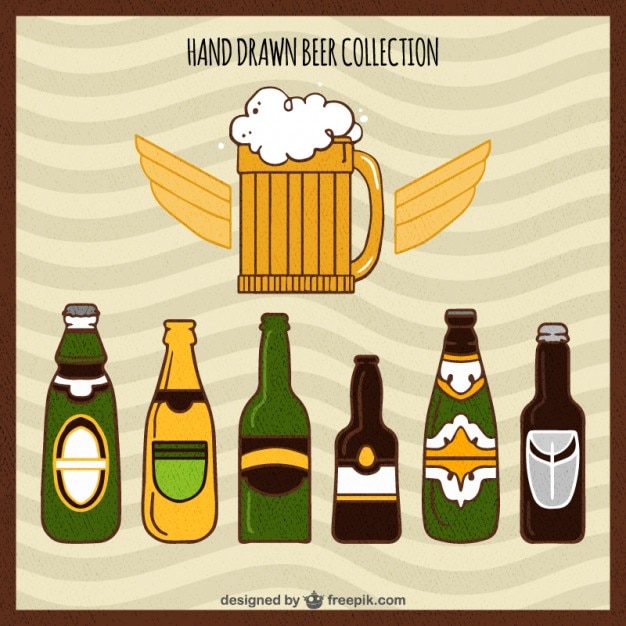This digital artwork features an array of hand-drawn beer illustrations against a tan or cream-colored backdrop, with subtle gray wave patterns. At the top, bold black text reads "Hand-Drawn Beer Collection." Below this title is a golden pint of beer crowned with white foam tumbling over the rim, flanked by slightly lighter golden wings. The bottom section of the image showcases six distinct beer bottles of various sizes and colors, including shades of forest green, yellow, lime green, amber brown, and dark brown. Each bottle sports a unique label and bottle cap design. The entire composition is framed by a thin brown border, and a note at the bottom credits the work to "designed by freepik.com."